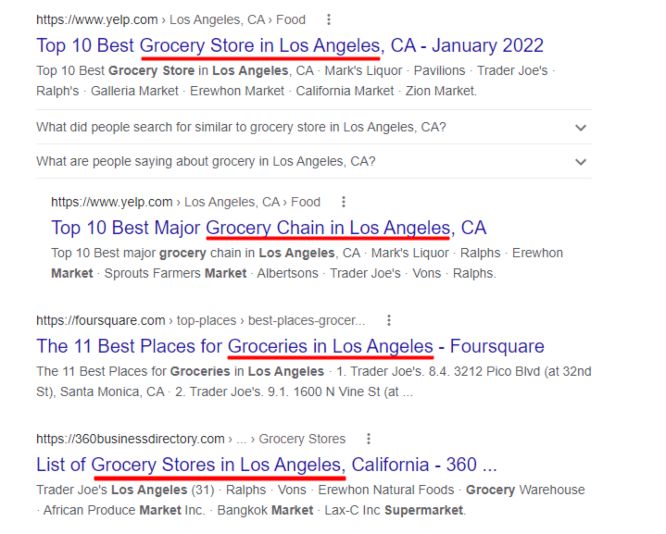The image displays the Google search results for "top 10 best grocery stores in Los Angeles, California" as of January 2022, according to Yelp.com. The results list prominent grocery stores including Mart's Liquor, Pavilion, Trader Joe's, Ralphs, Galleria Market, Erhu Han Market, California Market, and Zion Market. Below the list, there are additional questions such as "What do people search for similar to grocery stores in Los Angeles, California?" and "What are people saying about groceries in Los Angeles, California?" According to Yelp.com, the top 10 major grocery chains in Los Angeles also feature Mart's Liquor, Ralphs, Everthon Market, Sprouts Farmers Market, Albertsons, Trader Joe's, Vons, and Ralphs again. Additionally, a highlighted search result from Foursquare mentions Trader Joe's located at 3212 Pico Boulevard as one of the 11 best places for groceries in Los Angeles.